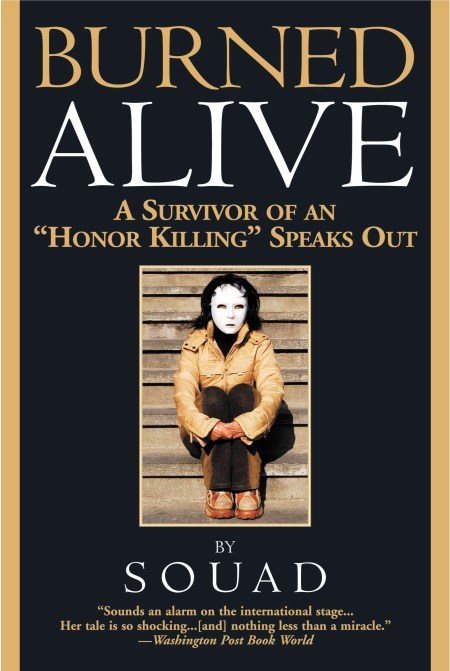The image depicts the cover of a book titled "Burned Alive: A Survivor of an Honor Killing Speaks Out" by Souad. The cover features a predominantly black background with thin yellow stripes running vertically along the left and right edges. Centrally, there is a striking photograph of a woman sitting on stone steps. She is garbed in a khaki jacket, brown pants, and brownish-red shoes. The woman, with black hair, is depicted wearing a white mask, characterized by openings for her eyes, nose, and mouth, reminiscent of a Halloween hockey mask. She clasps her hands around her knees, suggesting a protective or defensive posture. Notably, her hands appear mangled, hinting at the severity of her trauma. The title "Burned" is rendered in a tan hue, while "Alive" is white. The cover also features an endorsement from the Washington Post Book World, stating that Souad's tale "sounds an alarm on the international stage" and is "nothing less than a miracle," underscoring the gravity and significance of her story.